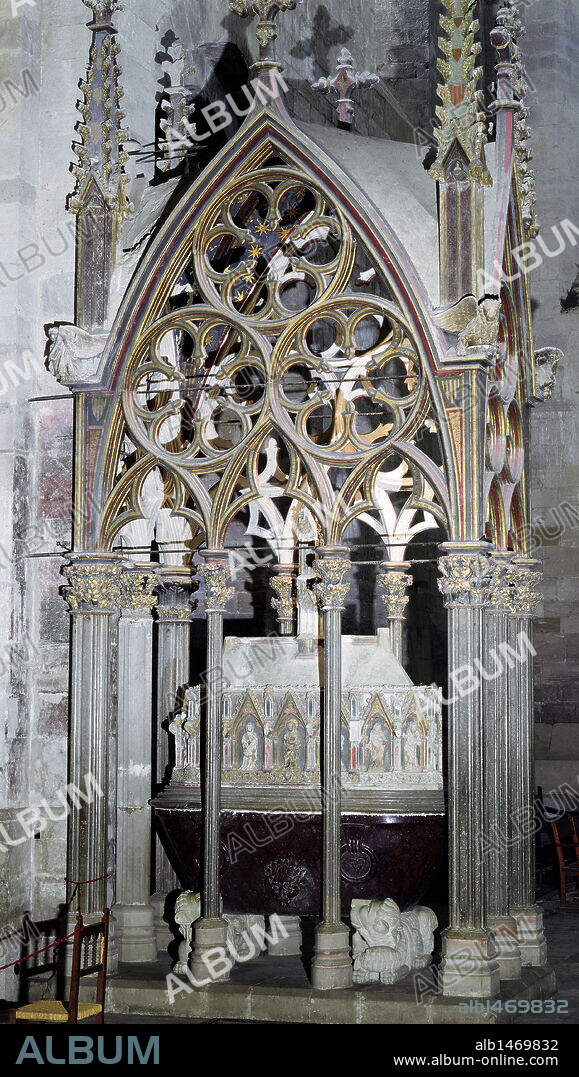The image depicts a vintage, ornate structure resembling a gazebo with metal poles, possibly situated in or near a church. The structure features a triangular top roof adorned with three circular murals or windows. Inside, detailed mural depictions include religious icons such as Jesus Christ and Mary. The entire image is rendered in color, with a light-colored diagonal watermark that reads "ALBUM" prominently displayed across it. The bottom left corner of the image displays "ALBUM" in blue against a black background, while the bottom right corner features the item number ALB1469832 and the website www.album-online.com. The structure also includes intricate posts and spires, adding to its elaborate design.